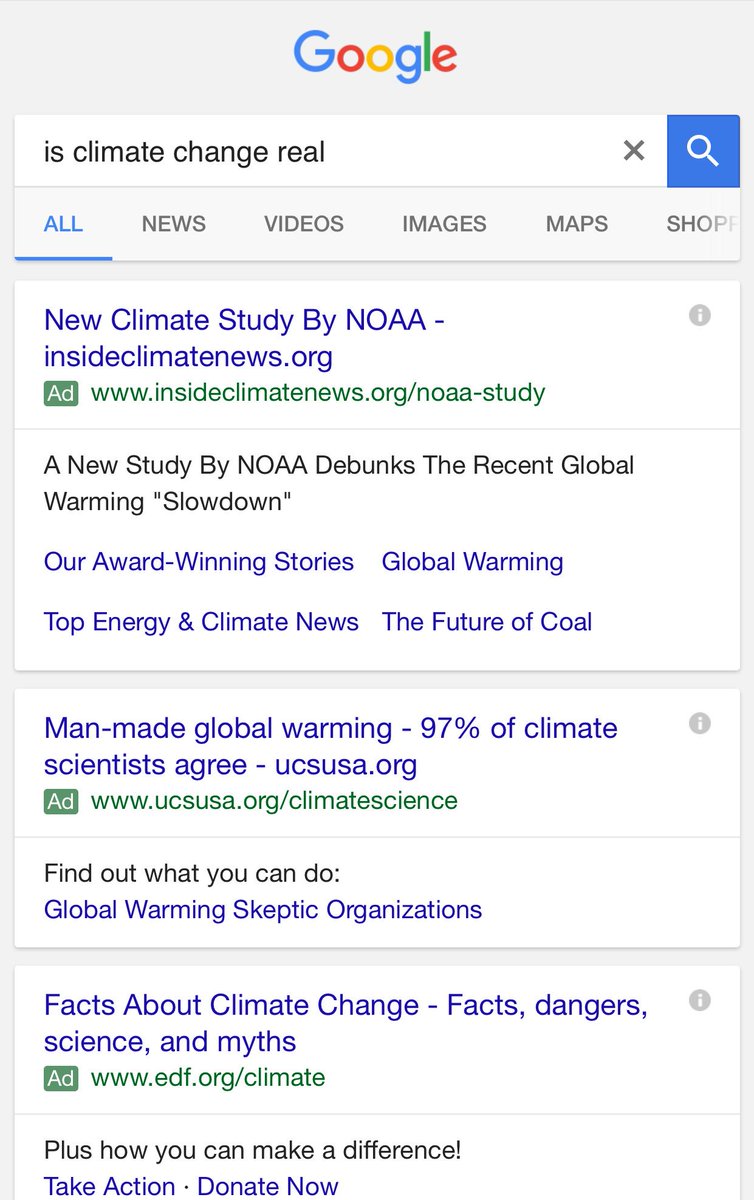The image depicts a Google search results page for the query "Is climate change real?" At the top, the search box prominently displays the query. Below it, there are various clickable links for different categories: "All," "News," "Videos," "Images," "Maps," and "Shopping."

The first section of the search results highlights a featured snippet from InsideClimateNews.org. The snippet, marked with a green "Ad" label, is titled "New Climate Study by N.O.A.A." The accompanying text, "A new study by N.O.A.A. debunks the recent global warming slowdown," suggests critical insights into current climate science. Further details mention, "Our award-winning stories, global warming, and top energy and climate news, the future of coal."

Following that, another result from UCSUSA.org, also highlighted in blue, states, "Man-made global warming: 97% of climate scientists agree." It is tagged with a green "Ad" label as well. Additional call-to-action content reads, "Find out what you can do," accompanied by a link that leads to information about "global warming skeptic organizations."

The next search result is a highlighted entry titled, "Facts about climate change: facts, dangers, science, and myths," indicating a comprehensive resource. Beneath it, a related advertisement from EDF.org, tagged in green, promotes climate action and information.

The final section of the page reads, "Plus how you can make a difference. Take action. Donate now," urging users towards proactive engagement.